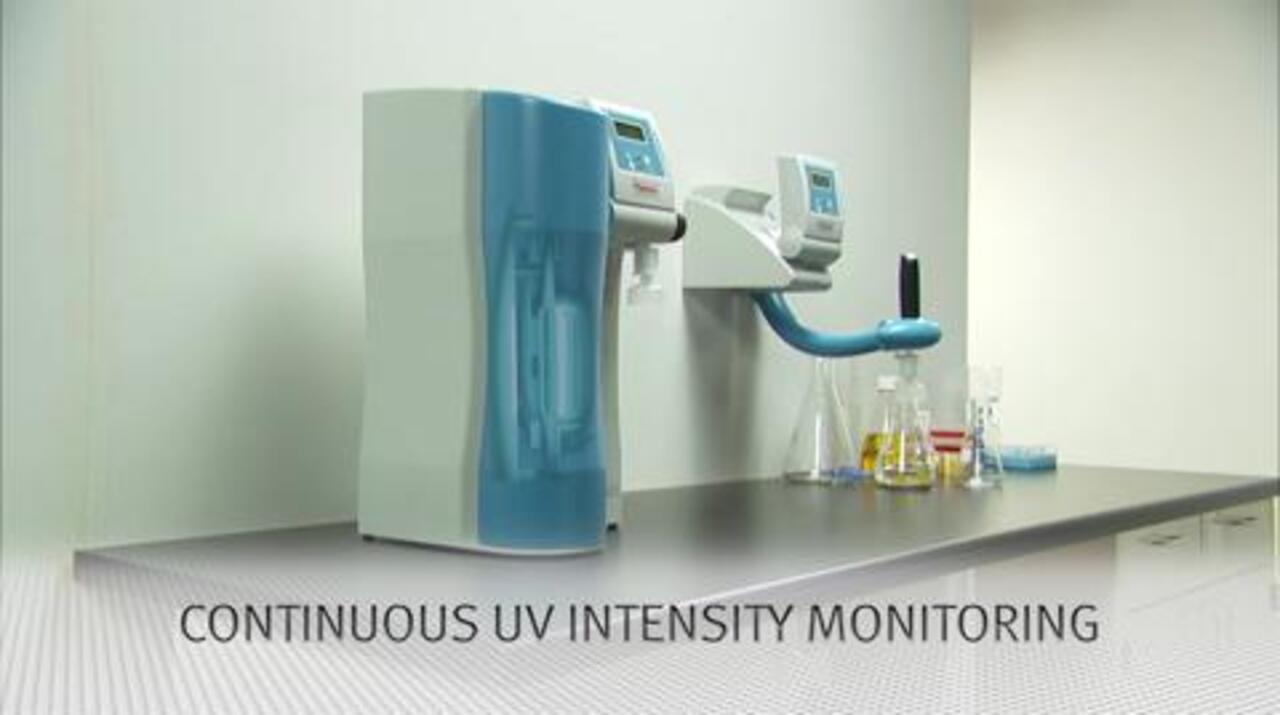Illustration of a Medical Workspace Featuring Continuous UV Intensity Monitoring

This detailed illustration, evocative of imagery featured in medical journals or websites, captures a clinical workspace designed for Continuous UV Intensity Monitoring. The setting is a stainless steel countertop, typical of medical environments, with visible drawers beneath and a clear leg space for seating. The scene is framed by plain white walls that converge in a corner, enhancing the sterile ambiance.

Prominently displayed on the counter is a printed title reading "Continuous UV Intensity Monitoring." The counter itself is occupied by two substantial pieces of equipment, one notably featuring a handle for ease of use. In the background, there are three or four beakers containing various liquids, along with a small plastic case, suggesting the presence of essential materials for medical or laboratory procedures. The overall setup underscores the meticulous nature of continuous monitoring in a professional healthcare setting.